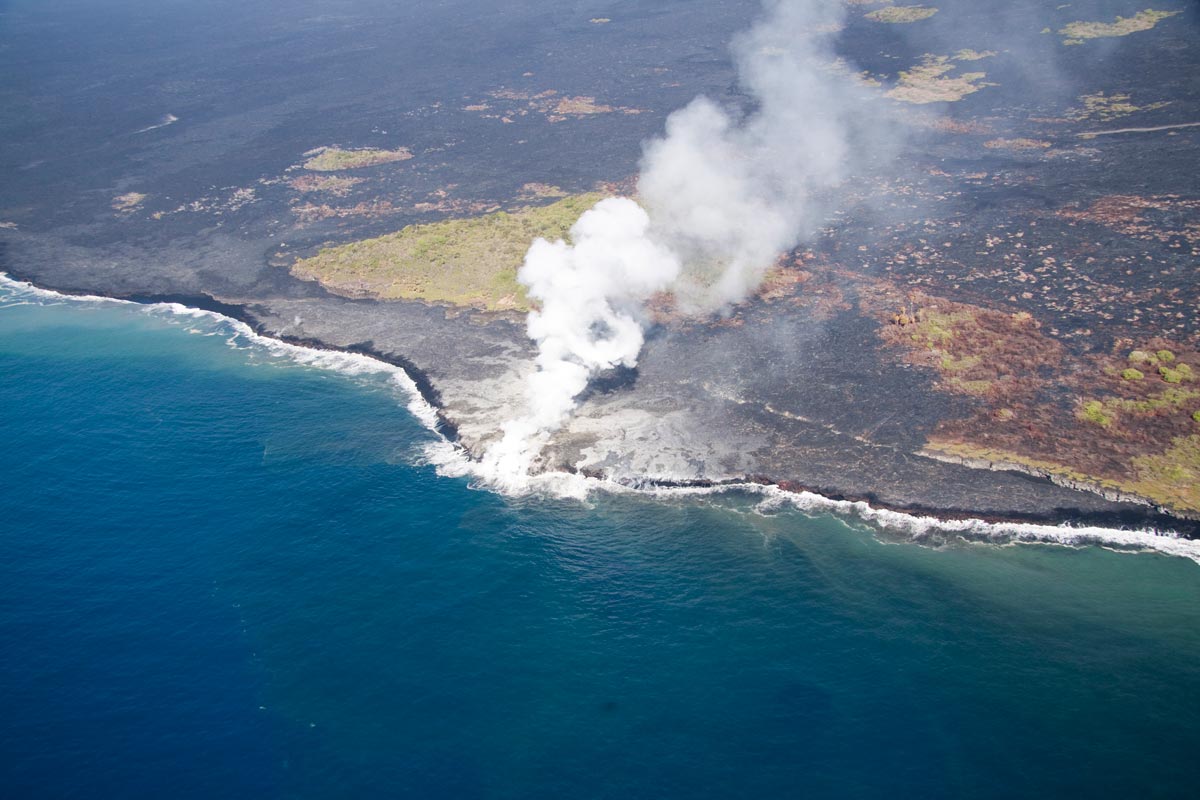An aerial photograph taken during the daytime shows a striking coastal scene where land meets water. The image is rectangular, approximately six inches wide by four inches high, and is likely captured from an airplane or drone. The bottom half of the photo is dominated by greenish-blue water, with white waves visibly crashing onto the shoreline. This shoreline forms a curved, downward angle from the upper left side to the lower right corner, creating a distinct border between the land and sea.

The upper half of the photograph features primarily brown and gray land, with patches of green, especially noticeable in the middle and on the right side. The land appears somewhat barren with signs of dead grass. Intriguingly, right at the juncture of land and water, in the central region, there are large plumes of white smoke ascending. These smoke clouds appear thick and voluminous, suggestive of volcanic activity or some intense combustible event. The smoke rises high, transitioning from white to shades of gray as it reaches the upper part of the image, adding a dramatic contrast against the natural colors of the land and water.